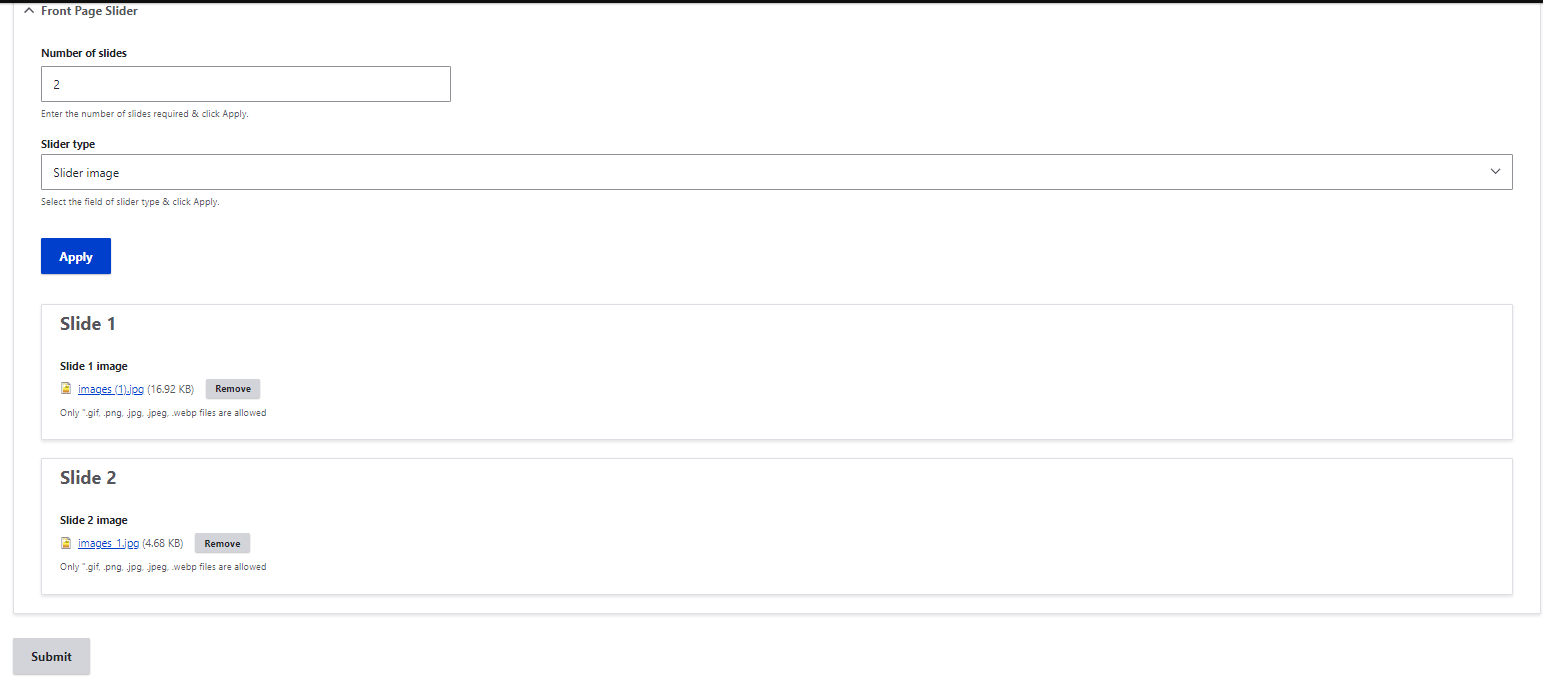The image displays a user interface for managing a front page slider. The top left corner features the label "Front Page Slider." Below this, elements are arranged vertically. The first element is "Number of Slides," accompanied by a rectangle containing the number "2." Next, "Slider Type" and "Slider Image" are listed, followed by an unreadable short sentence.

Further down, there is an "Apply" button within a blue square. The section below includes "Slide 1," with options to add an image file highlighted in blue and remove it in gray. "Slide 2" mirrors these options. At the bottom left, a light gray square contains the word "Submit" in black. A horizontal black line runs across the top of the image. The entire interface is set against a white background.